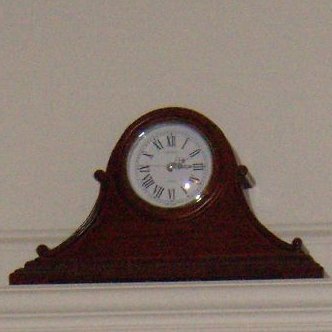This photograph captures an elegant, old-fashioned mantel clock situated indoors. The clock rests on a white shelf, which seamlessly blends with the white wall behind it. A wooden border, possibly part of a fireplace mantle or trim, is visible in front of the shelf. The clock itself is crafted from dark brown wood, featuring a rectangular base that extends upward into a rounded top. The clock's face is encased in a glass covering, showcasing a white background adorned with black Roman numerals. Silver hands add a refined contrast to the dial, though their exact positions cannot be discerned. The overall design emphasizes an antique aesthetic, meticulously blending functional and decorative elements.